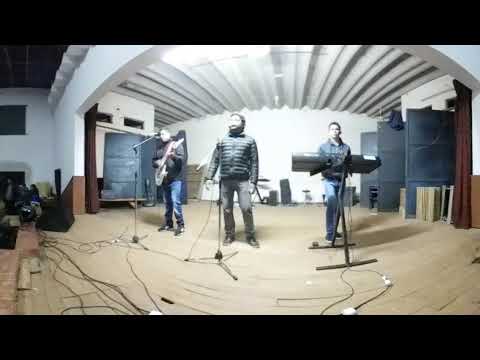In this interior stage setting with a beige ground and a white ceiling crisscrossed by horizontal pylons, three men are engaged in a musical performance. The back wall is white and flanked by open grey metal doors on both the left and right sides of the stage. At center stage, a man wearing a black puffer jacket and grey long pants stands in front of a microphone. To his left, a man in blue jeans and a black jacket also has a microphone stand and is holding a guitar. On the right, another man, clad in jeans, is positioned behind an electronic piano or synthesizer. The stage is adorned with fluorescent strips on the ceiling, which light up the scene. The setting has numerous cords scattered around, contributing to a rough and unfinished atmosphere, suggesting ongoing preparations or a practice session rather than an official performance. The photograph appears to be taken with a fisheye lens or at a distorted angle to encapsulate the entire setup, hinting at the span and depth of the room.